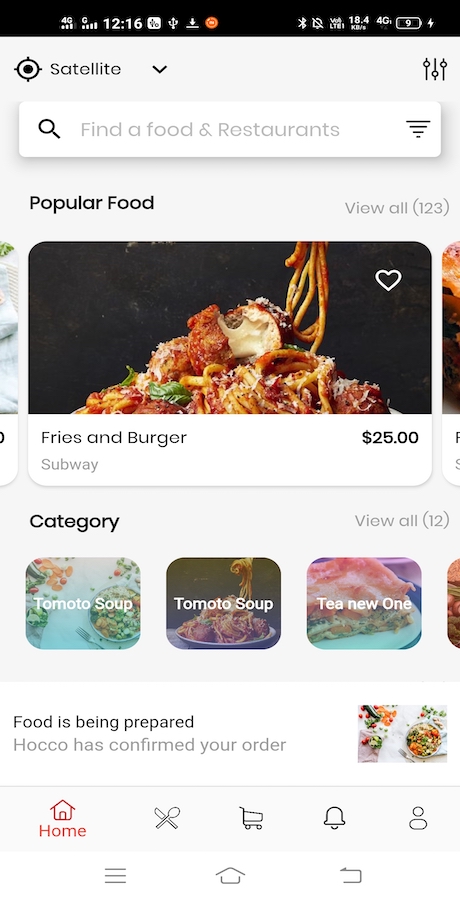**Detailed Caption:**

This screenshot is from a food delivery app displayed on a smartphone. The top inch of the screen is black, housing vital status icons. On the left side, about an inch in, various connectivity and status indicators can be seen: '4G' is displayed first, followed by three white bars, then the letter 'G', and below it, four additional bars. Adjacent to these, on the right, is the time '12:16'. 

Further to the right, there's a small white square containing obscure black details, alongside a white candlestick-like icon with an arrow pointing downwards beneath it, accompanied by a red circle featuring a red robot head. On the far right of this black bar are a lightning bolt icon, a battery icon, a '9', '4G', '18.4 kbps', 'LTE', and icons indicating silence mode and Bluetooth connectivity.

Below this black bar, the screen transitions to a light grayish-blue color. On the left side, there's a scope-like circle icon, next to which the word 'Satellite' is written in black, followed by a down-pointing greater-than symbol.

Directly beneath this segment is a white search bar stretching horizontally across the screen. Below the search bar, in black text, it reads 'Popular Food', while on the right-hand side, there is a designation of 'You All (1, 2, 3)'. Below this label is an image where the background is predominantly black, featuring a plate of spaghetti and meatballs.

The screen then shows another section; on the left side, it lists 'Fries and Burger', and on the right side, a price of '$25'. Beneath 'Fries', in gray text, the word 'Subway' is written. Underneath this, the text 'Category' is displayed, accompanied by three images of food items. The first image is labeled 'White Tomato Soup', the second simply 'Tomato Soup' in white text, and the last 'Tea New' also in white text.

Finally, there's additional navigational information about the restaurant: home page, shopping cart, notifications, and other icons typically found at the bottom of an app interface.